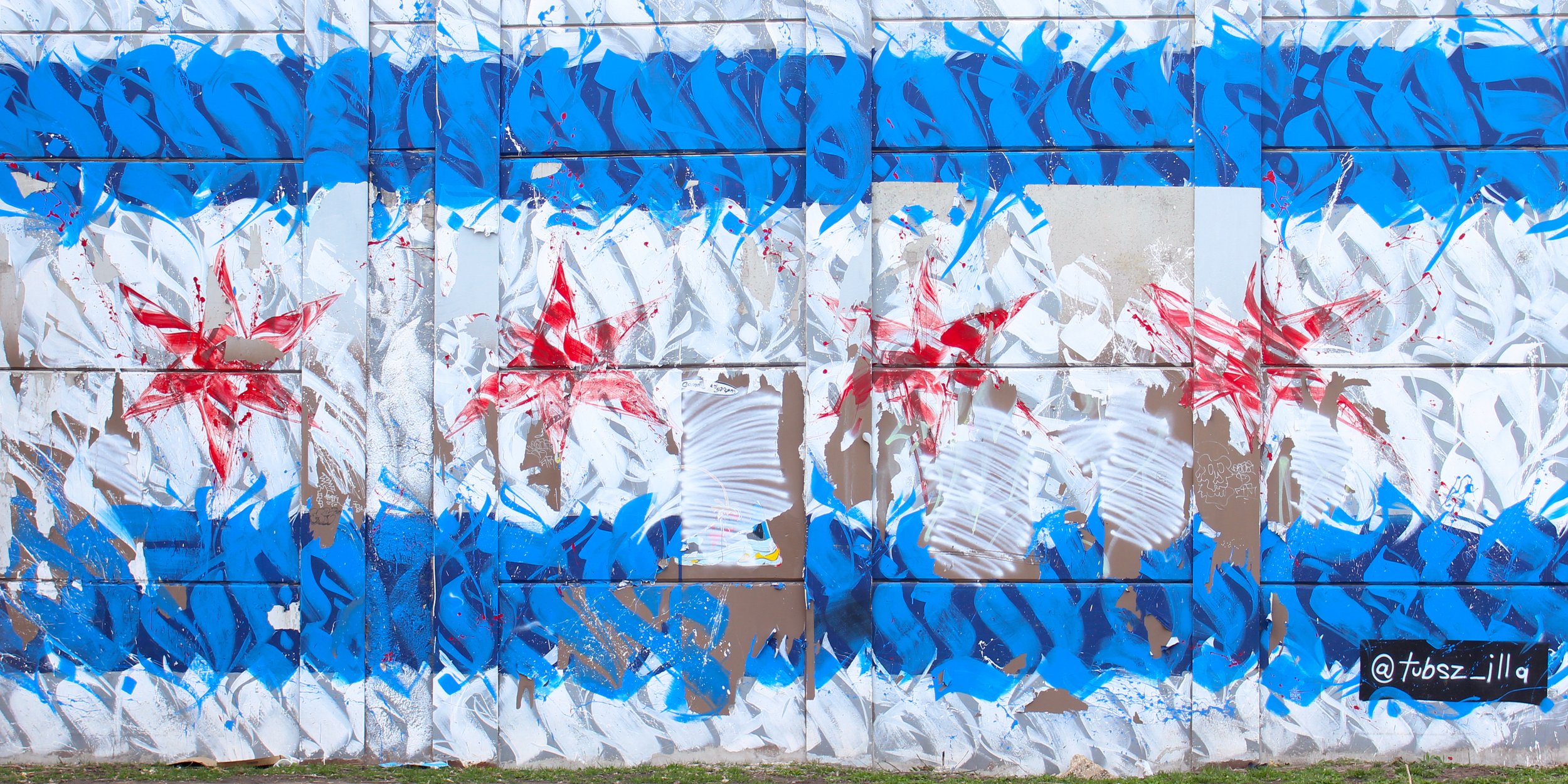This detailed image depicts the Chicago flag painted on a textured surface that resembles ribbon or cut newspaper. The flag has horizontal stripes beginning with a white band at the top, followed by a light blue stripe, then another white band in the middle. In the central white stripe, there are four red stars, each partially visible and having a ribbon-like texture. Below this, another light blue stripe appears, followed by yet another white stripe. The texture and coloration give a faded, almost handcrafted appearance to the flag. In the bottom right corner of the image, there is a black rectangle with white text that reads "@TUBSC_ILLA".